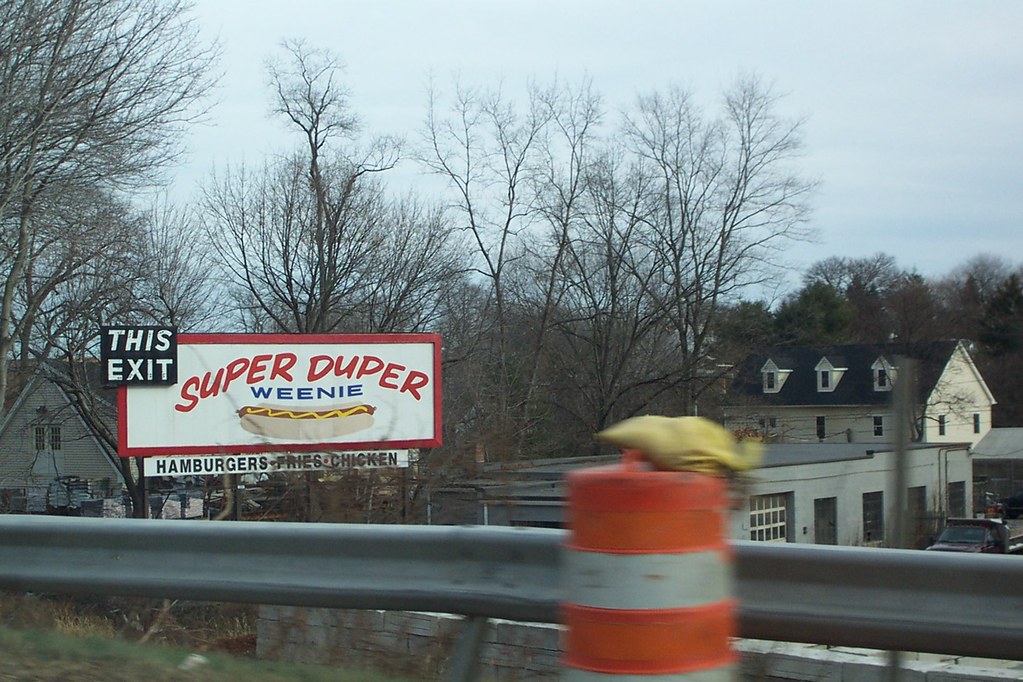Captured from the perspective of a car window while driving on the highway, this photo vividly showcases the side of a freeway. On the immediate right, metal guardrails are prominently visible, typical of freeway boundaries. A bright orange traffic cone stands nearby, adding a pop of color to the scene. In the background, a cluster of buildings can be seen, hinting at nearby urban life. A large, eye-catching road sign is also visible, humorously advertising an exit that leads to "Super Duper Weenie." The sign features an image of a hot dog and lists a variety of menu items including burgers, hamburgers, fries, and chicken. The combination of these elements encapsulates a fleeting yet detailed snapshot of roadside Americana.